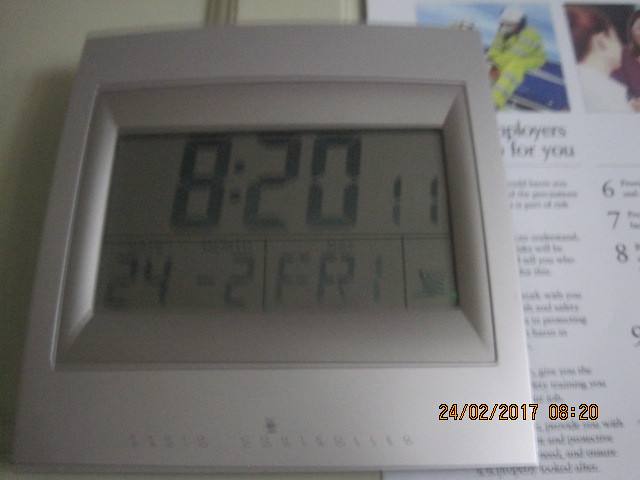The image depicts a gray, rectangular room thermometer prominently displaying various readings. The digital screen presents the time as 8:20 and 11 seconds. Below the time, it shows the date formatted as "24-2," possibly indicating February 24th, and the day of the week as "Friday." There's also a small, unclear icon that resembles a tiny box, making its purpose difficult to decipher. The brand or manufacturer of the thermometer is not visible in the image. The photograph was taken on February 24, 2017, at 8:20 AM, as indicated by an overlay on the image. The thermometer, with its uniform color scheme and structured design featuring an inner and an outer box, is placed on an open magazine page that contains various numbers and text, adding a backdrop of printed material to the scene.